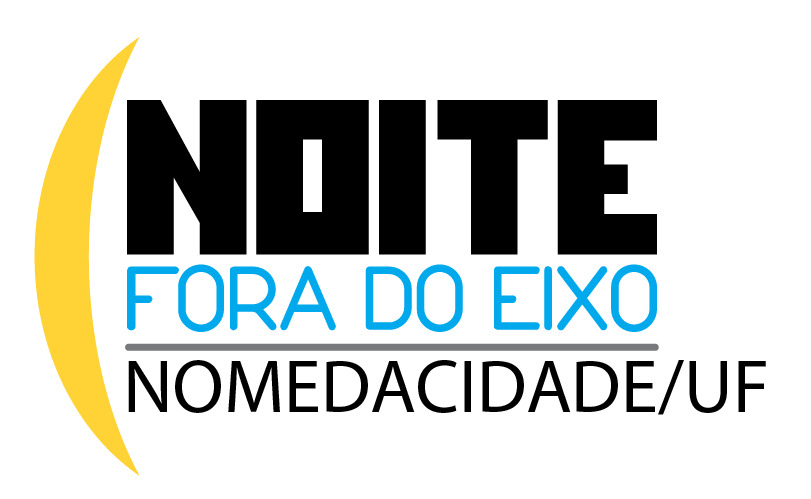The image depicts a simple yet striking logo against a white background. On the left, there's a yellow crescent moon shape. To its right, in bold black block letters, the text reads "N-O-I-T-E". Below this, in smaller but capitalized light blue letters, are the words "F-O-R-A D-O E-I-X-O". Just underneath, separated by a light gray line, is the additional text "N-O-M-E-D-A-C-I-D-A-D-E / U-F" in black. The design skillfully integrates elements of typography and subtle color illustration to create a clean, informative logo in a foreign language.